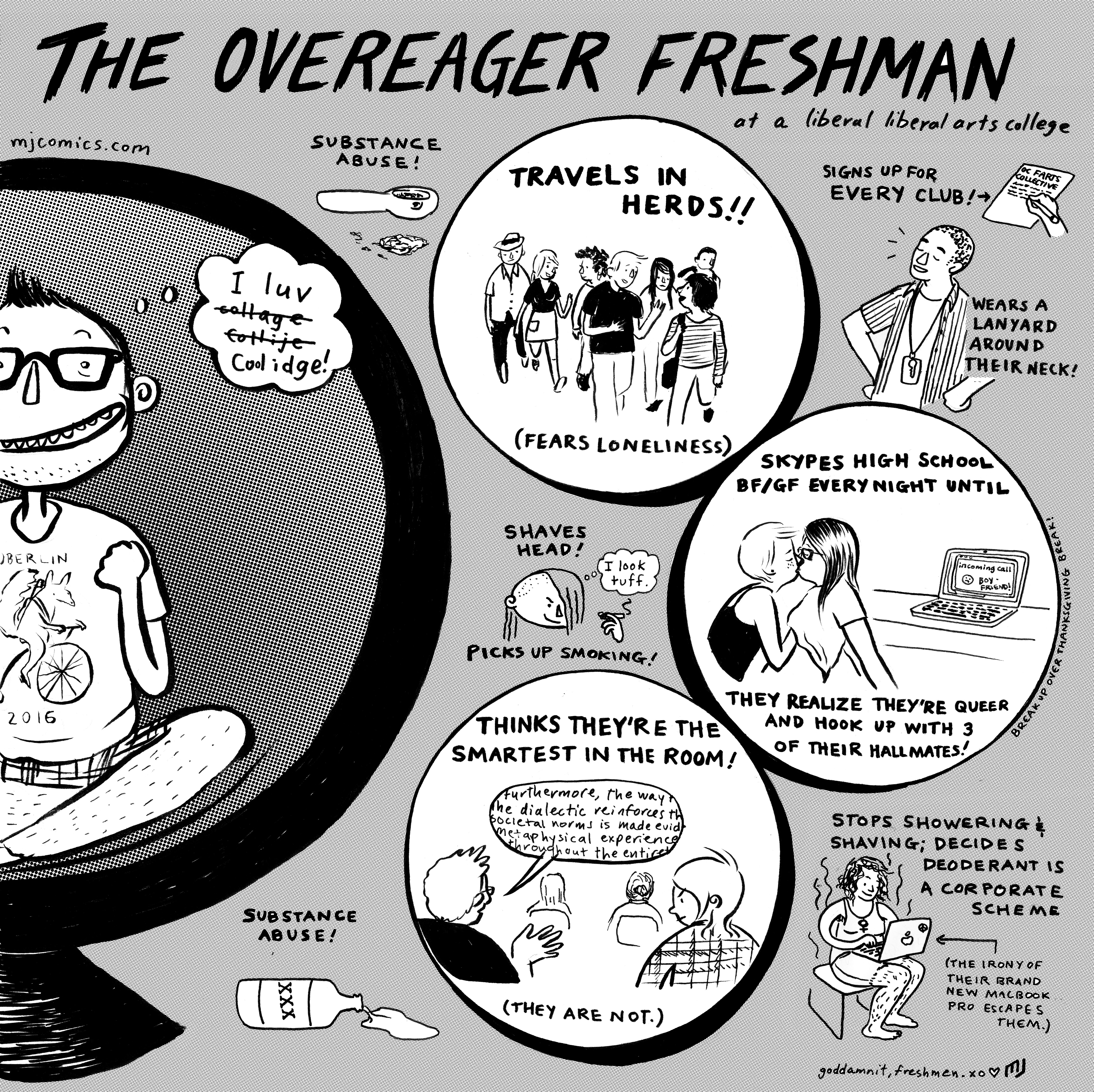The detailed, cleaned-up caption for the image would be:

"This is a handwritten pamphlet or poster titled 'The Over-Eager Freshman' in bold black capital letters across the top. Below the title are several white circles containing illustrations and text detailing various behaviors. In the top circle, labeled 'Travels in Herds (Fears Loneliness),' there is a drawing of a group of young people walking together. Another circle, located to the right, shows an illustration of two people kissing with the caption 'Skypes high school boyfriend/girlfriend every night until they realize they're queer and hook up with three of their hallmates.' To the left, there's a larger circle featuring a person sitting inside it, grinning broadly, with a thought bubble that reads, 'I love college,' though misspelled. This person is described as wearing glasses, having a bicycle, and a shirt with '2016' on it, portraying the freshman who thinks they are the smartest in the room but are not. Scattered around the pamphlet are additional smaller drawings, including one of a spilled bottle labeled 'Substance Abuse,' pictures promoting conspiracy theories about not showering or shaving to save deodorant, and another of a person holding a laptop. Overall, it humorously depicts the quirks and behaviors of an over-eager freshman at a liberal arts college."